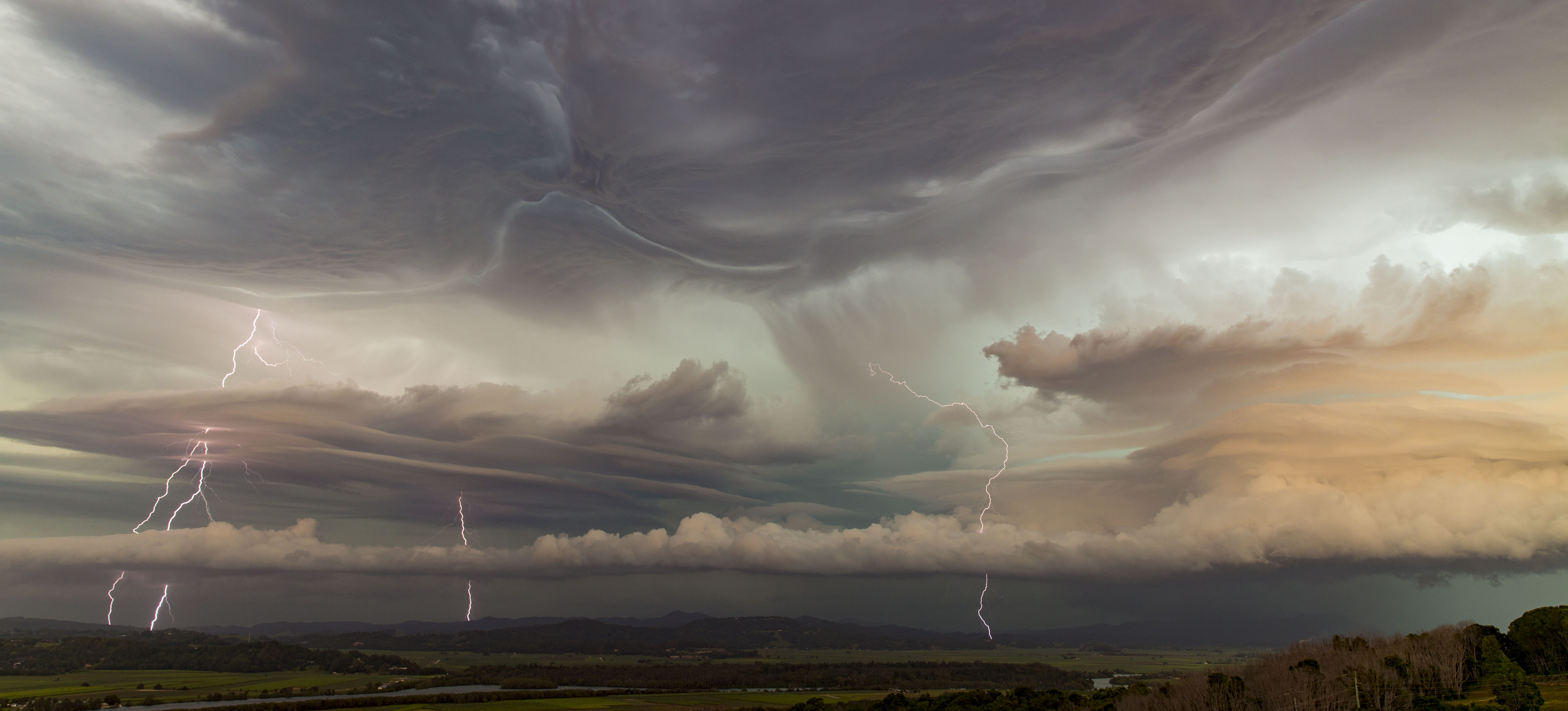A soft-colored photograph, almost reminiscent of a painting, captures a dramatic dark sky scene. Dominating 90-95% of the frame, the sky is menacingly beautiful, filled with large clouds and pierced by multiple streaks of lightning. The horizon is faintly visible at the bottom, giving way to what appears to be a stormy sea—a grey expanse that seamlessly merges with the tumultuous sky due to the lack of reflection from the lightning. At the very bottom, dark patches of greenery and a cliff face on the right hint at a rugged, bog-like landscape unique to Ireland.

The sky is filled with several massive clouds, including a prominent round one near the top. Towards the left, a lighter patch of sky allows vivid bolts of lightning to descend, illuminating a pink and green-toned cloud beneath. In the middle, more lightning strikes, casting an otherworldly green glow. On the right, amidst a concentration of white light from the lightning, an orange cloud catches the illumination, hovering ominously just above the cliff. The detailed interplay of colors and light creates an ethereal, almost surreal atmosphere in this dramatic natural scene.